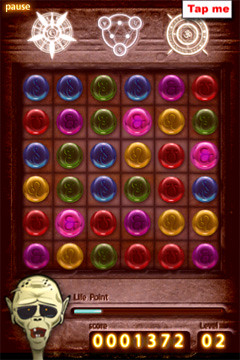The image captures a paused video game scene with a low-resolution, grainy appearance and muted colors. In the upper left corner, the word "pause" is displayed in small yellow sans-serif font. On the right side, a white triangle features the red text "tap me." The bottom left corner showcases a stylized creature - potentially a ghoul, zombie, or skull - with a bulbous head, narrow jaw, open mouth, and sunken black eyes.

The game board is displayed prominently with a current score of 1,372 points at level 2. The board consists of regular square shapes, filled with 3D-effect colored circles in blue, green, pink, red, yellow, and orange, each featuring a brighter outer rim and a darker inner rim. Above these circles is a horizontal band with a woodgrain texture that holds three white, sketched images resembling compass roses or actual compasses.